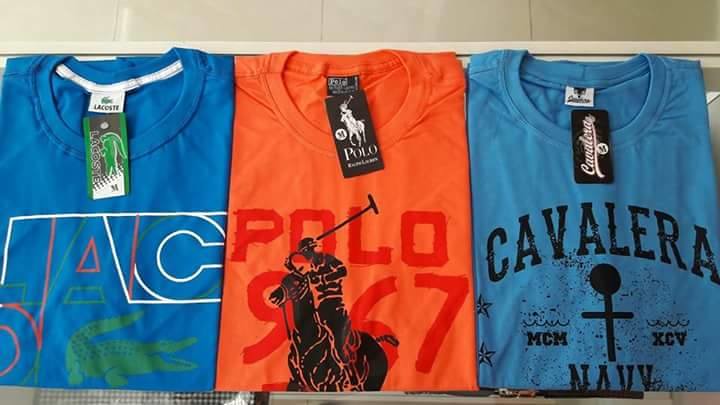This photograph showcases a neatly folded display of three medium-sized t-shirts, arranged side-by-side on a white tiled floor, each sporting distinct graphics and tags. The leftmost t-shirt, a dark blue Lacoste, features thin white, pink, and green lines forming the letters "AC," accompanied by the iconic green alligator logo, which has its tail up and mouth open, facing right. This shirt also has a multi-colored tag sticking out from the collar. The middle t-shirt is bright orange, branded by Polo, with the text "Polo 967" in red, alongside a black silhouette of a polo player on horseback facing left, with his polo stick raised high. This shirt also includes a black and white rectangular tag at the collar. The t-shirt on the right, a lighter blue Cavalera, displays the word "CAVALERA" in a prominent arch, along with the text "MCM XCV," a cross shape with a circle at the top, and the partially visible word "Navy" beneath the fold. This shirt also sports a black and white rectangular tag at the collar.